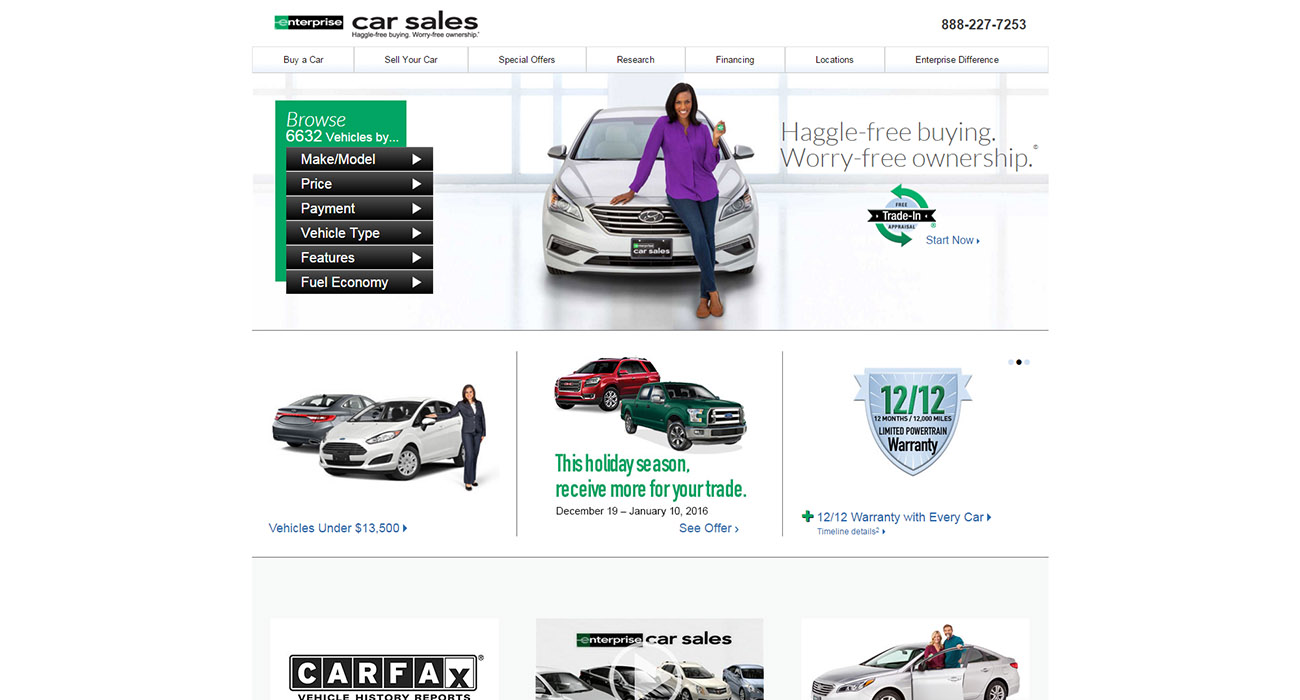The image is from Enterprise, with the logo prominently displayed at the top. The logo features the word "enterprise" in lowercase on a black background, accompanied by a shaded green "e." Beneath the logo, the text reads: "Car Sales, Haggle-Free Buying, Worry-Free Ownership."

In the header, there are various navigation options including “Buy Car,” “Sell Your Car,” “Special Offers,” “Research,” “Financing,” “Locations,” and “Enterprise Difference.” At the top-right corner, a contact number is visible: 888-227-7253.

To the left, there are nine smaller images structured in three rows. The top section invites users to browse through 6,632 vehicles and includes dropdown menus for "Make," "Model," "Price," "Payment," "Vehicle Type," "Features," and "Fuel Economy.”

Adjacent to this, an image features a woman with dark skin sitting on a gray car. She wears a purple top, blue pants, and brown shoes. The accompanying text says: "Haggle-Free Buying, Worry-Free Ownership," along with a prompt for a trade-in and free appraisal: “Start Now.”

Below, there are three horizontal boxes:
1. **Vehicles Under $13,500**: Two cars—a white one and a gray one—are showcased. A woman in a dark gray pantsuit points to the white car.
2. **Holiday Offer**: The center box highlights a holiday trade-in offer available from December 19. Two vehicles—a green truck and a red van—are displayed.
3. **Warranty Information**: A shield symbol with “12 out of 12” denotes the 12 months/12,000 miles limited powertrain warranty provided with every car.

At the bottom, there’s a segment on Carfax Vehicle History Reports. A clickable video link titled “Enterprise Car Sales” features four cars. Additionally, two people are pictured standing in front of a white compact car with the door open.

The layout and comprehensive information emphasize Enterprise's focus on a transparent, hassle-free car buying experience with reassuring after-sales guarantees.